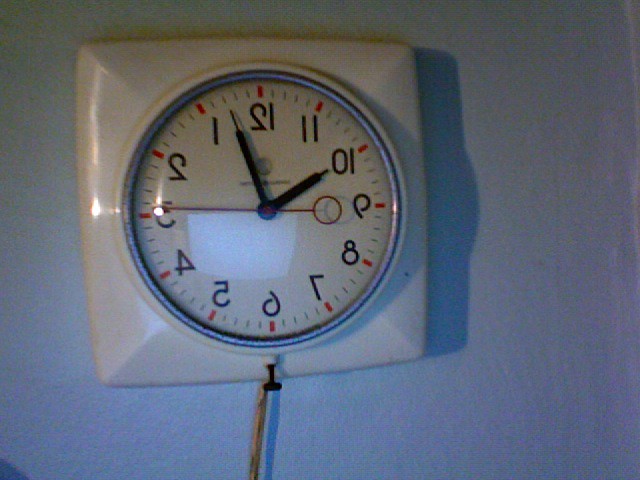This photograph depicts a wall clock with a unique feature: its numbers are arranged in reverse, with the 9 on the right and the 3 on the left, suggesting it's a backwards clock. The clock has a white face and is surrounded by a square white border, creating a clean, monochromatic appearance against the white wall it hangs on. The numbering is in black, with red markings for individual seconds. The clock has three hands: the hour and minute hands are black, while the second hand is a thin red line with a pointed end and a circle on the opposite end. The clock's surface is slightly reflective, hinting at a dim light source from the left, possibly a camera flash, creating a shadow to the right. Additionally, there is a winding knob below the 6 and an electric cord extending out from the bottom. The image quality is somewhat poor - blurry and low resolution - further enhanced by the faint shadow cast by the clock.